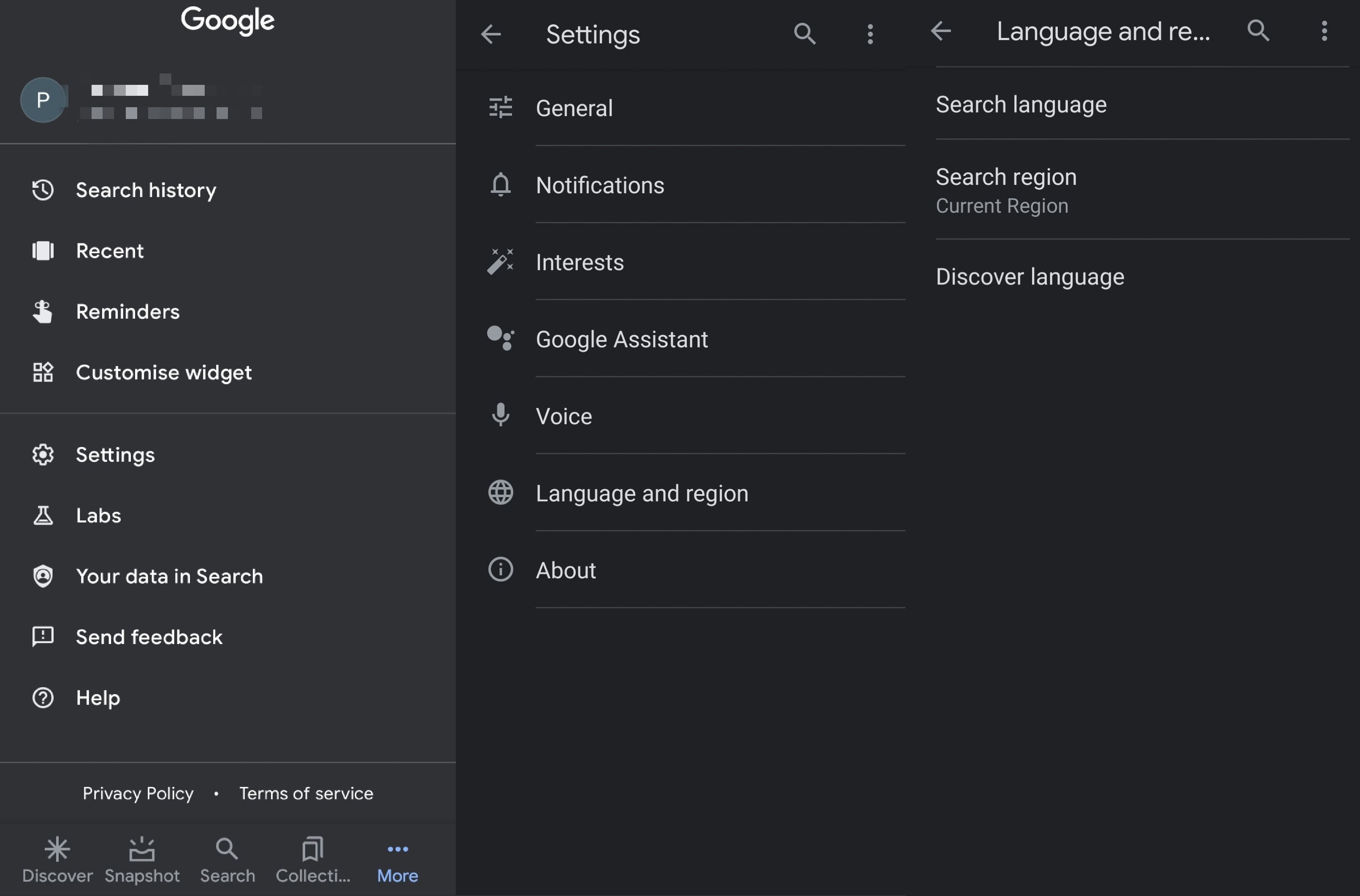The image displays a screenshot of a Google application interface on a smartphone. The background is black, providing a stark contrast to the white text and icons. On the left side of the screen, "Google" is prominently displayed in white. The user's profile icon features a gray circle with a white letter "P" in the center.

The screenshot includes various sections such as search history, recent, reminders, customized widget, settings, labs (represented by a beaker icon), and "Your data in Search," indicated by a crest. Additionally, there is a help section accessible through a button marked with a question mark, and privacy policies along with terms of service are also mentioned.

At the bottom of the interface, there are several tabs: "Discover" (denoted by a sun icon), "Snapshot," "Search" (indicated by a magnifying glass), "Collections," and "More," the latter written in blue font.

The central part of the screenshot focuses on the settings menu, which includes options such as general settings, notifications, interests, Google Assistant, voice, language and region (indicated by a globe icon), and an "About" section (marked with an informational icon).

A subsequent screenshot within the interface shows language settings, featuring options to search for a language, set a search region for the current language, and select a discover language button.